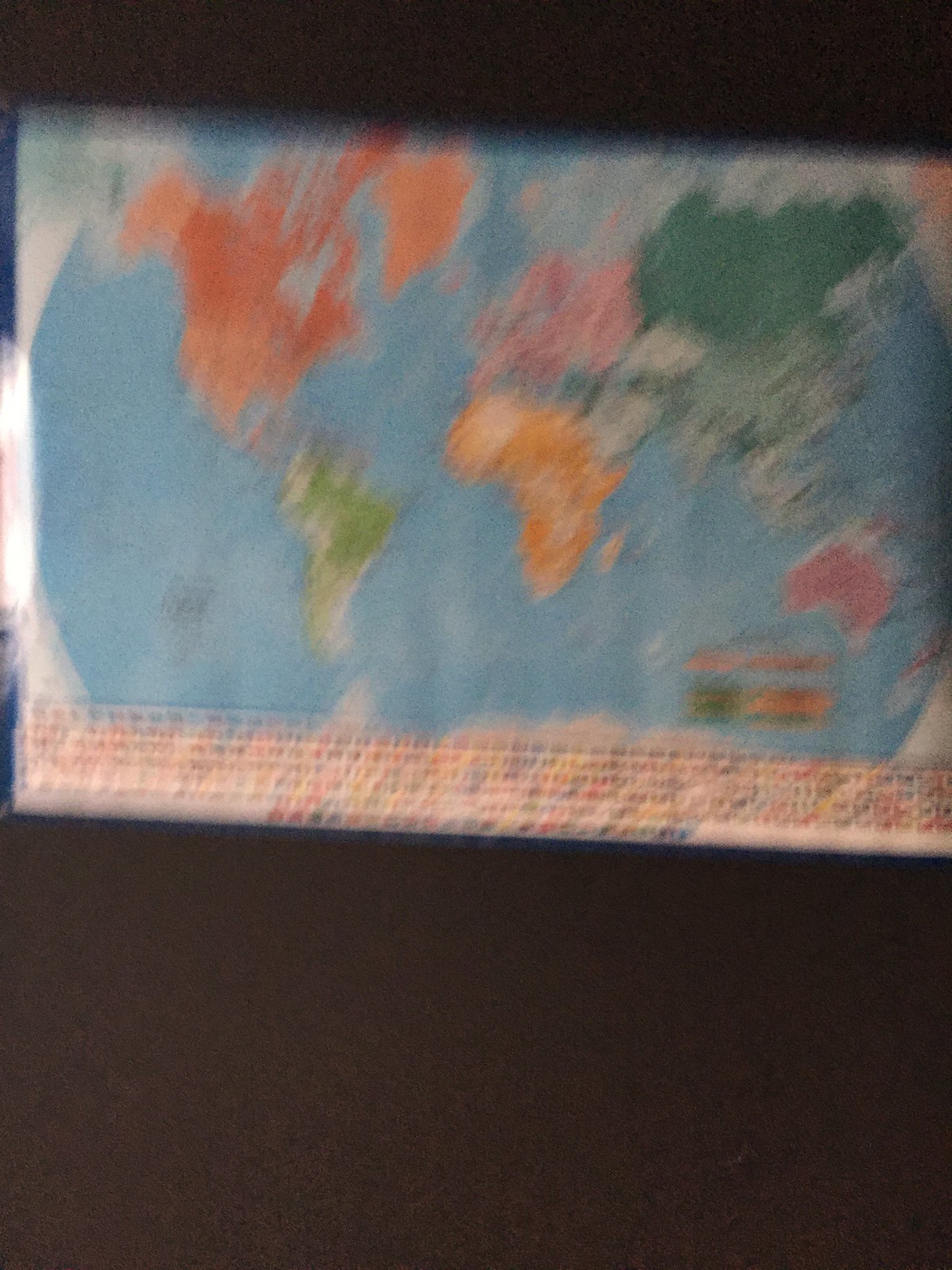This image is a very blurry photograph of a rectangular, flat world map set against a gray background. The map prominently features the light blue color of the oceans, while the continents are depicted in a spectrum of colors including dark orange, light orange, green, white, teal, dark green, pink, and darker pink. North America is tinted red, South America appears greenish, Africa is orange, Europe is shaded in a light pink, Asia is mostly dark green, and Australia is pinkish. The bottom of the map shows a mosaic pattern composed of blurred colored squares in shades of orange, yellow, green, blue, purple, and pink. Additionally, there is unreadable text at the bottom, and the map is bordered by a solid black strip on the top and a slightly larger black strip on the bottom. The overall blurriness makes it difficult to discern any further details or the material of the map.